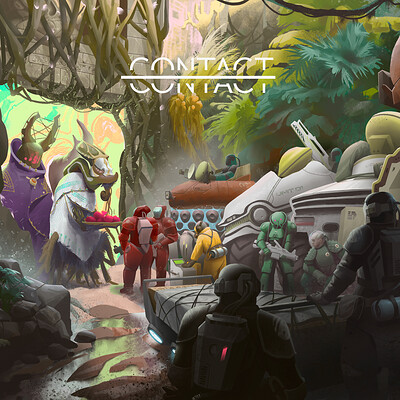The highly detailed and evocative image is a futuristic, sci-fi themed drawing or painting. The scene is populated by characters that resemble astronauts or soldiers, outfitted in large, intricate suits or spacesuits. Central to the composition are two large, alien-like creatures that dominate the space with their imposing figures and unique features. One creature is adorned with a purple robe and has intertwined strings between two antler-like horns, with red slashes across the front of its head. The other creature, towering above the others, sports a single prominent horn on its forehead with a smaller one trailing behind, clutching a plate filled with red orbs. 

In the middle left, the aliens appear to be emerging from a doorway, standing out starkly due to their height compared to the humanoids around them. To the right, two gray, tank-like machines can be seen, with two people positioned atop them and another two standing in the foreground, facing the tanks. The background is dense with trees, vines, and indeterminate machinery, encapsulating the scene in an otherworldly forest-like setting.

Prominently displayed towards the top center of the image is the word "CONTACT" in white text, segmented by a horizontal white line running through the letters. Behind this text, the environment broadens to reveal more walls with vines and plants, emphasizing the intertwining of the mechanical and natural world. This intricate and bustling scene vividly brings to life an alien encounter in a richly detailed sci-fi milieu.